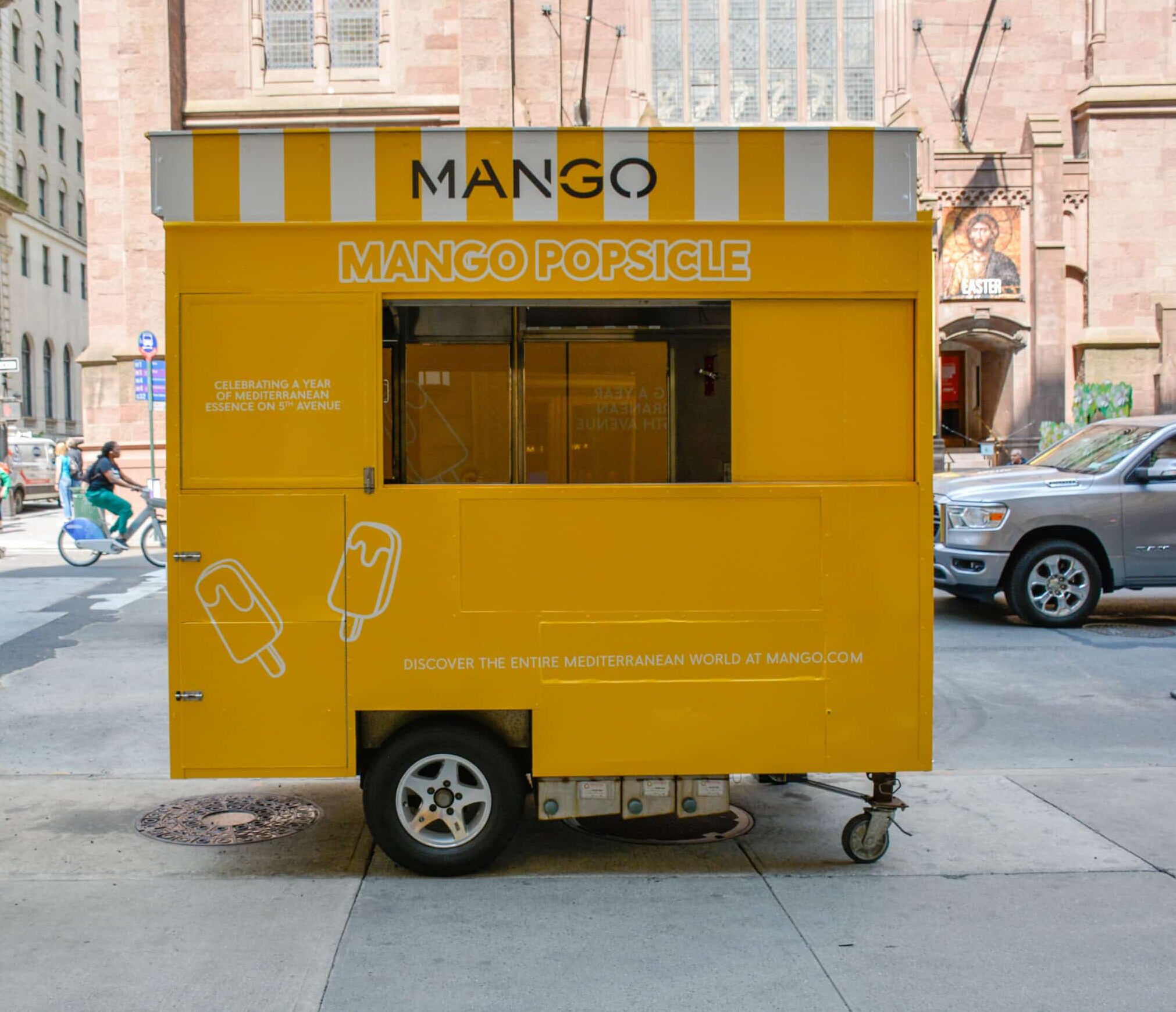The image depicts a vibrant, orange food cart set against a bustling city backdrop, positioned in a parking lot with cars and a bicyclist nearby. The cart, designed for selling mango popsicles, features an eye-catching, striped orange and white banner with the word "MANGO" in bold black letters at the top. Directly under this, "Mango Popsicle" is prominently displayed in bright orange text with a white outline on the cart's body. On the lower right-hand corner of the cart, there are artistic depictions of popsicles, outlined in white against the orange background. An open dispensing window is visible, although there are no vendors present at the moment. Inside, the space appears to be stocked with boxes, possibly keeping the popsicles cold, suggesting a refrigerated interior. Additionally, a slogan reads: "Celebrating a year of Mediterranean essence on Fifth Avenue. Discover the entire Mediterranean world at mango.com," adding a touch of marketing flair to the cart's vibrant presence. The entire setup is mounted on wheels, indicating mobility, but is currently stationary.